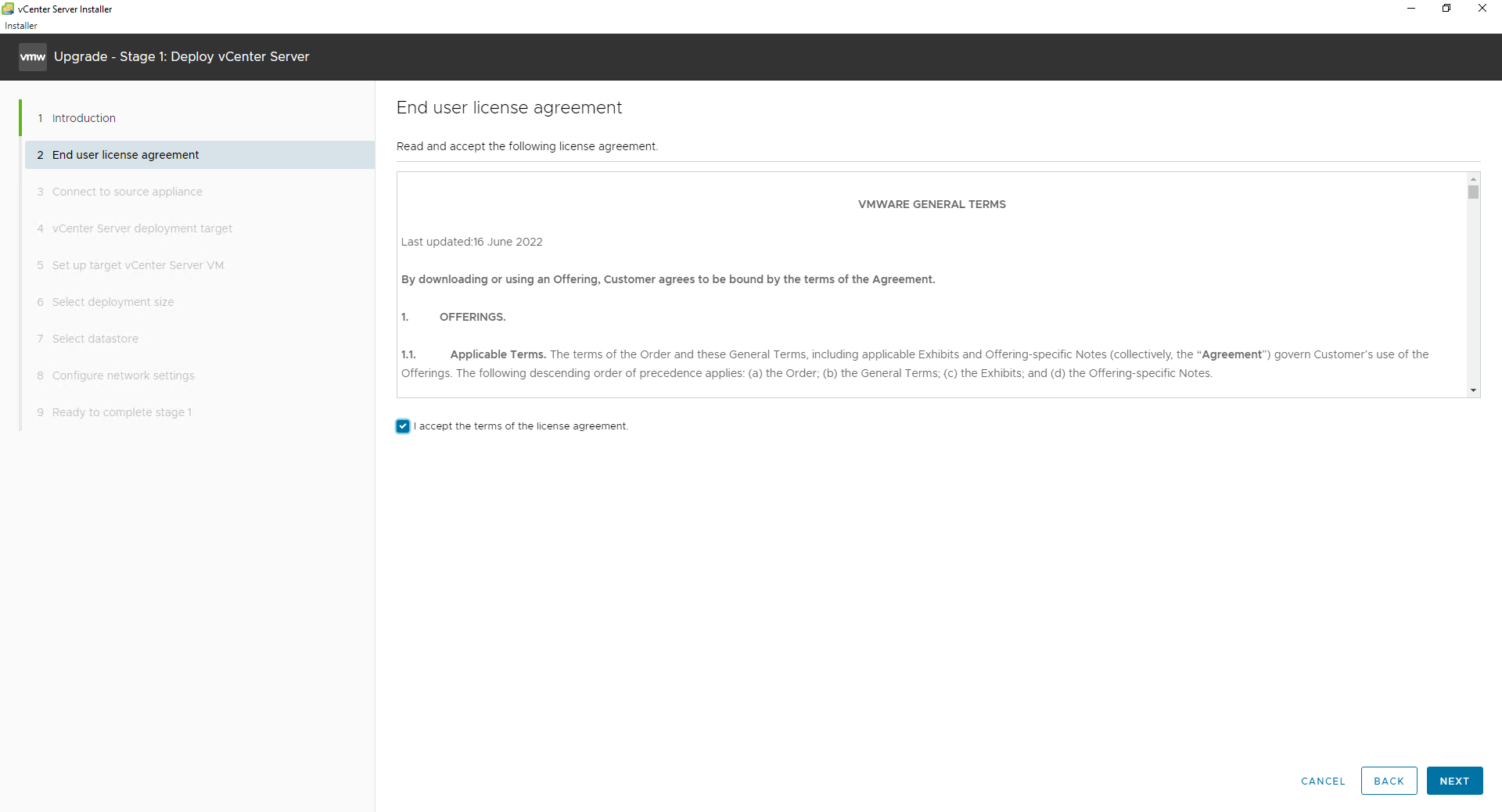This detailed screenshot is captured from an application running on a Windows 10 operating system, evident by the sharp, rectangular window borders—a distinguishing feature from Windows 11. On the far left of the screenshot, the title "vCenter Service Installer" is prominently displayed along with its emblem. On the far right, the familiar minimize, maximize, and close buttons for the window are visible.

Near the top left of the interface, the caption "Upgrade Stage 1: Deploy vCenter Server" is clearly marked. The installer is structured into nine steps, with Step 1 (Introduction) already completed. The current focus is on Step 2, dealing with the End User License Agreement (EULA).

Centrally, the page reiterates "End User License Agreement," followed by the directive to "Read and Accept the Following License Agreements," particularly highlighting VMware's General Terms. Below these terms, there is a pre-checked dialogue box indicating acceptance of the license agreement terms. At the bottom right of the screen, a "Next" button is available for the user to click and proceed to the subsequent steps of the installation process.